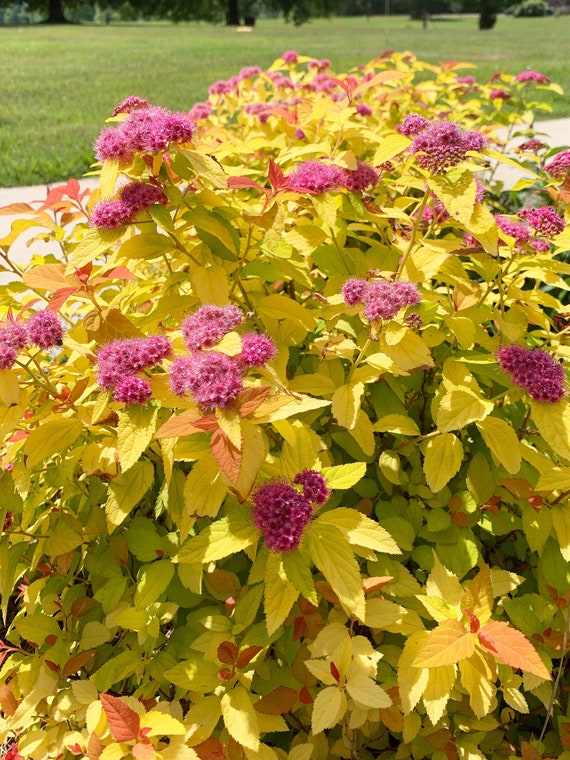This detailed image captures a vibrant outdoor scene on a bright, sunny day. In the foreground, a large flowering bush, likely a spirea, displays an array of brilliant yellow leaves mingled with some green, suggesting that yellow is the primary blooming color. The bush features clusters of flowers with a mix of purplish-pink petals and darker centers, creating a striking contrast against the foliage. The bush itself has an intriguing, rounded shape that emerges from the ground. Behind the flowers, a long stretch of green grass extends, bordered by a variety of skinny evergreen trees. Additionally, a single walkway cuts through the background, further enhancing the sense of a well-maintained park or residential area. This combination of elements, from the vivid colors of the flowers to the lush greenery and structured pathway, creates a serene and picturesque natural setting.